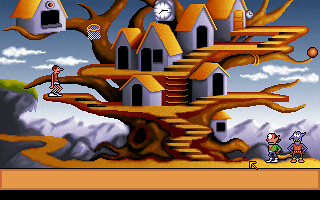In this vibrant and lively video game scene, a whimsical tree house stands prominently against a backdrop of towering mountains, fluffy clouds, and a clear sky. The tree house, rooted in a sturdy brown trunk, features charming yellow roofs and white walls, creating a cozy and inviting atmosphere. A basketball hoop is attached to the tree house, adding a playful touch. On the lower level, a path flanked by lush greenery leads to the black steps reaching up to the tree house. Along these steps, two characters are positioned on the right side, presumably making their way upwards. Another character is seen on the second level of the tree house, to the left, adding to the dynamic feel of the scene. The left side of the background showcases additional trees and a meandering path through the greenery. A rustic clock is also mounted on the tree, emphasizing the intricate details that make this setting enchanting. Despite the lack of any specific game-related markers or numbers, the image clearly captures the essence of a fantastical game world brimming with adventure and charm.